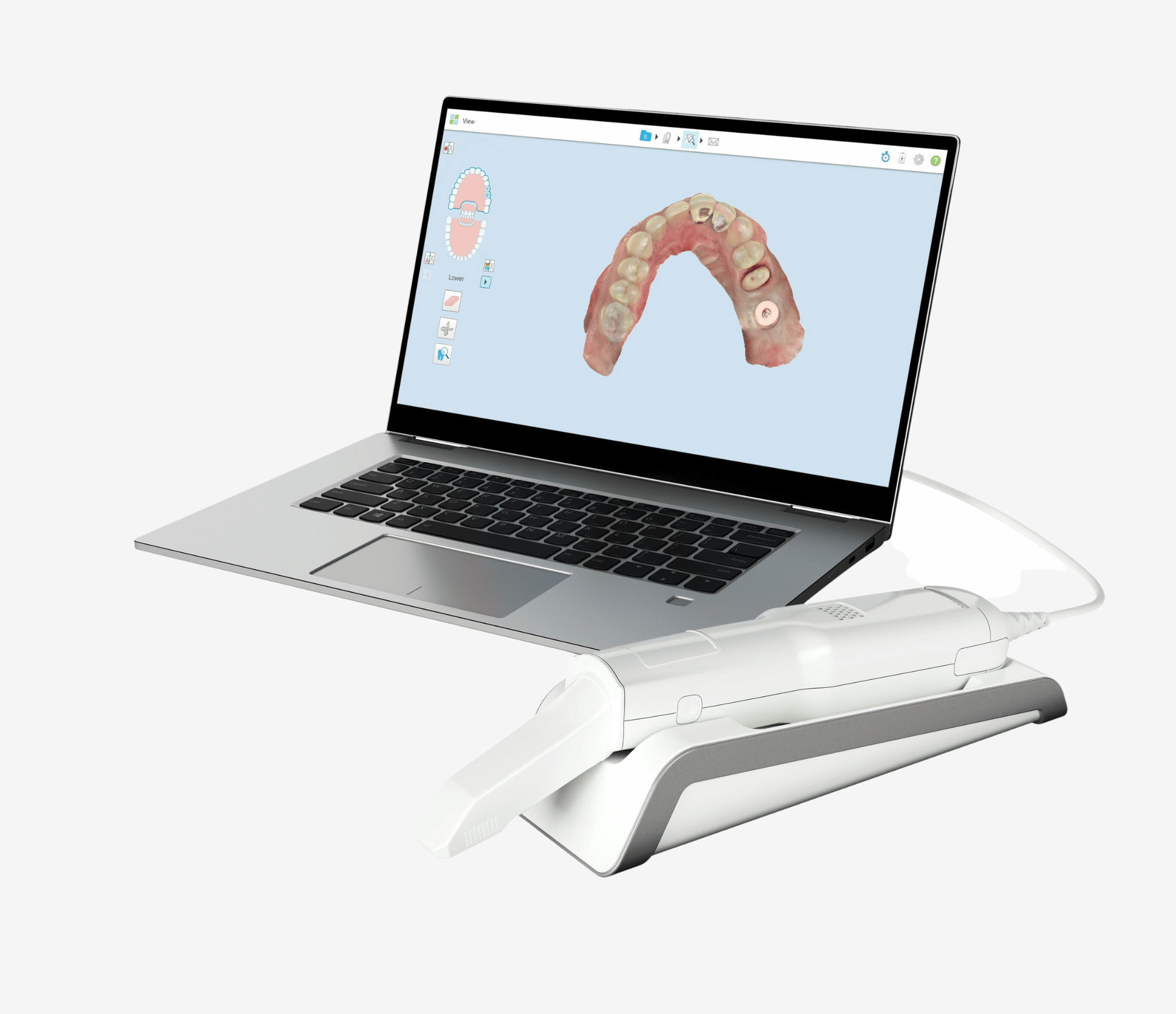The image depicts a photograph of a laptop with a silvery gray chrome body and solid black keys, bordered by a black frame around the monitor. On the laptop screen is a detailed computer-generated image of a mouth with visible teeth, some of which appear to have dental issues, possibly with one spot circled. Adjacent to the main image, on the left, are a couple of illustrated images likely showing a reference for the close-up. To the lower right of the laptop screen rests a sleek, cylindrical white device with a slightly curved edge, connected to the laptop via a cord extending from its back. This device, reminiscent of dental tools used for treatments like fillings, is sitting on a gray and white holder, implying that it is charging or being stored when not in use. The entire setup suggests the image relates to a dental technology or procedure, perhaps showcasing a tool for dental diagnostics or treatments.